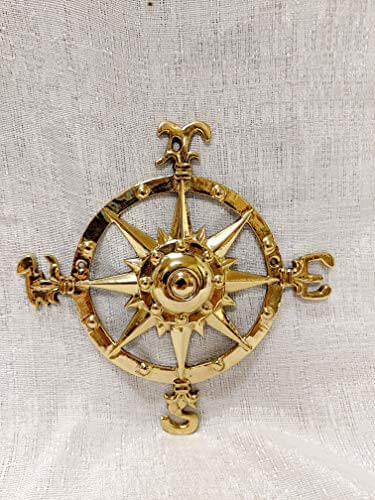The image depicts a golden brooch in the shape of a compass, resting on a thin, white cloth background that transitions to a grayish hue towards the top. The brooch features an intricate design with an outer ring adorned with diamonds. Prominently displayed on the ring are the directional letters—N for North at the top, E for East on the right, S for South at the bottom, and W for West on the left. At the center of the compass is an eight-pointed star that resembles a sun, with some tips coinciding with the directional points and smaller points in between. The star is connected to the outer ring, housing a central knob and several small metal circles within. The entire piece is crafted from shiny, gold-plated metal, exuding a radiant luster. This detailed object could function as a brooch or a pendant, with potential attachment points suggested by a possible pin on the back or a small hole for threading a chain.